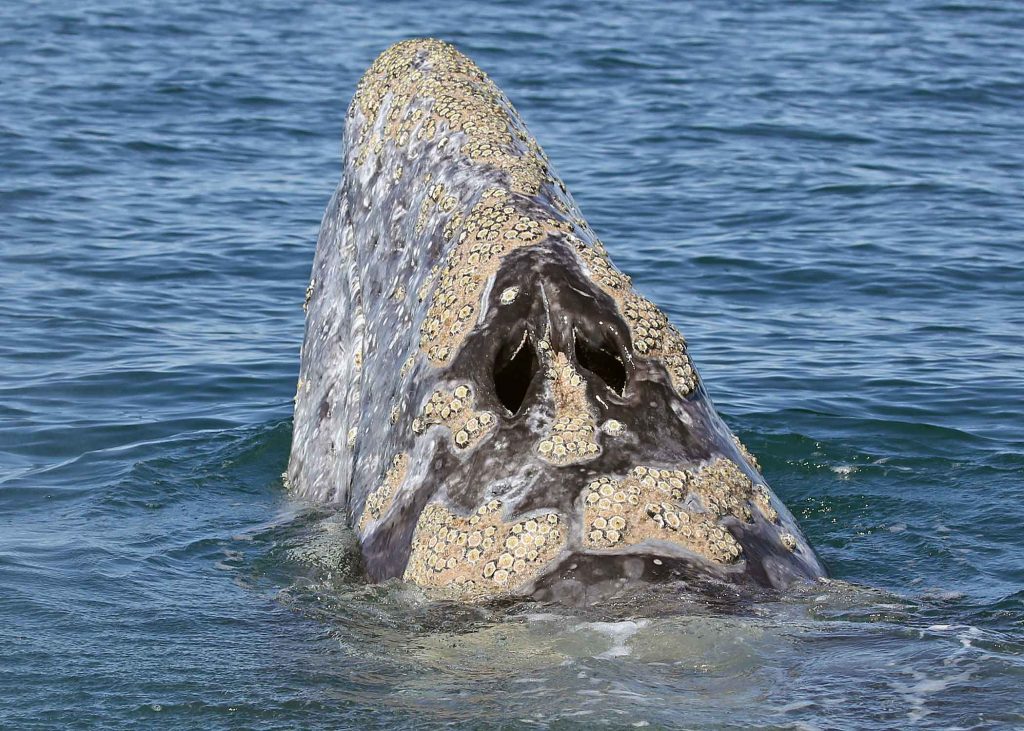In this outdoor daytime photograph, the dark blue ocean with gentle ripples dominates the background, creating a vast and serene marine backdrop. Emerging from the water is the head of a gray whale, distinctly adorned with light brown barnacle-like patterns. The whale's back is black, contrasting starkly with the barnacle textures that cover its hump. Prominently visible on top of its head are two blowholes, giving an illusion of eyes, although the actual eyes of the whale are not visible. There are no people or text in the image, emphasizing the solitary and majestic appearance of the whale breaching through the calm water.